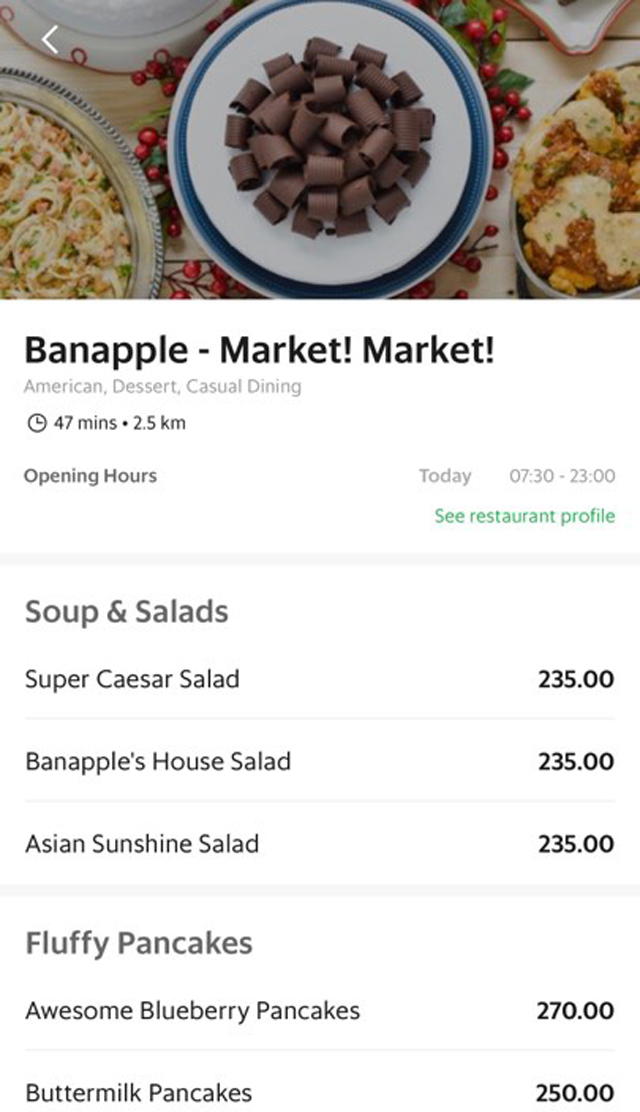The photograph appears to be a top-down view of a menu, showcasing a selection of dishes and information from a casual dining restaurant. The main parts of the image are described as follows:

At the top of the image, there is a round plate with intricate chocolate swirls on it. The plate is predominantly white, with a blue border. On the left side of the photo, partially cut off, is a pasta dish. On the right side, there appears to be a dish featuring cheese and a brown sauce.

Beneath these dishes, in bold black font, there is text that reads, "Banana Apple" stylized as "B-A-N-A-P-P-L-E," followed by an exclamatory punctuation sequence. Below this, in non-bold gray text, the phrase "American dessert casual dining" is visible.

Further down, a black clock icon is accompanied by the text "47 minutes," suggesting a waiting time. Below this, "2.5 KM" is displayed, possibly indicating the distance of the restaurant from the current location. Continuing downwards, the restaurant's opening hours are listed in light gray text, showing "Today, 07.30-23.00." In green text below that, "C restaurant profile" invites viewers to explore more about the establishment.

A gray border separates the sections of the menu. In the next segment, gray text labels "Soups and Salads," which includes items such as "Super Caesar Salad," "Banana's House Salad," and "Asian Sunshine Salad." The prices for these items, listed in black, are each "235.00" in an unspecified currency.

Another gray border denotes the next section: "Fluffy Pancakes," which offers options like "Blueberry Pancakes" and "Buttermilk Pancakes." The prices listed beside them are "270.00" and "250.00," respectively.

This detailed menu layout combines culinary and logistical information to give potential diners a comprehensive overview of their dining options, prices, and operational details.